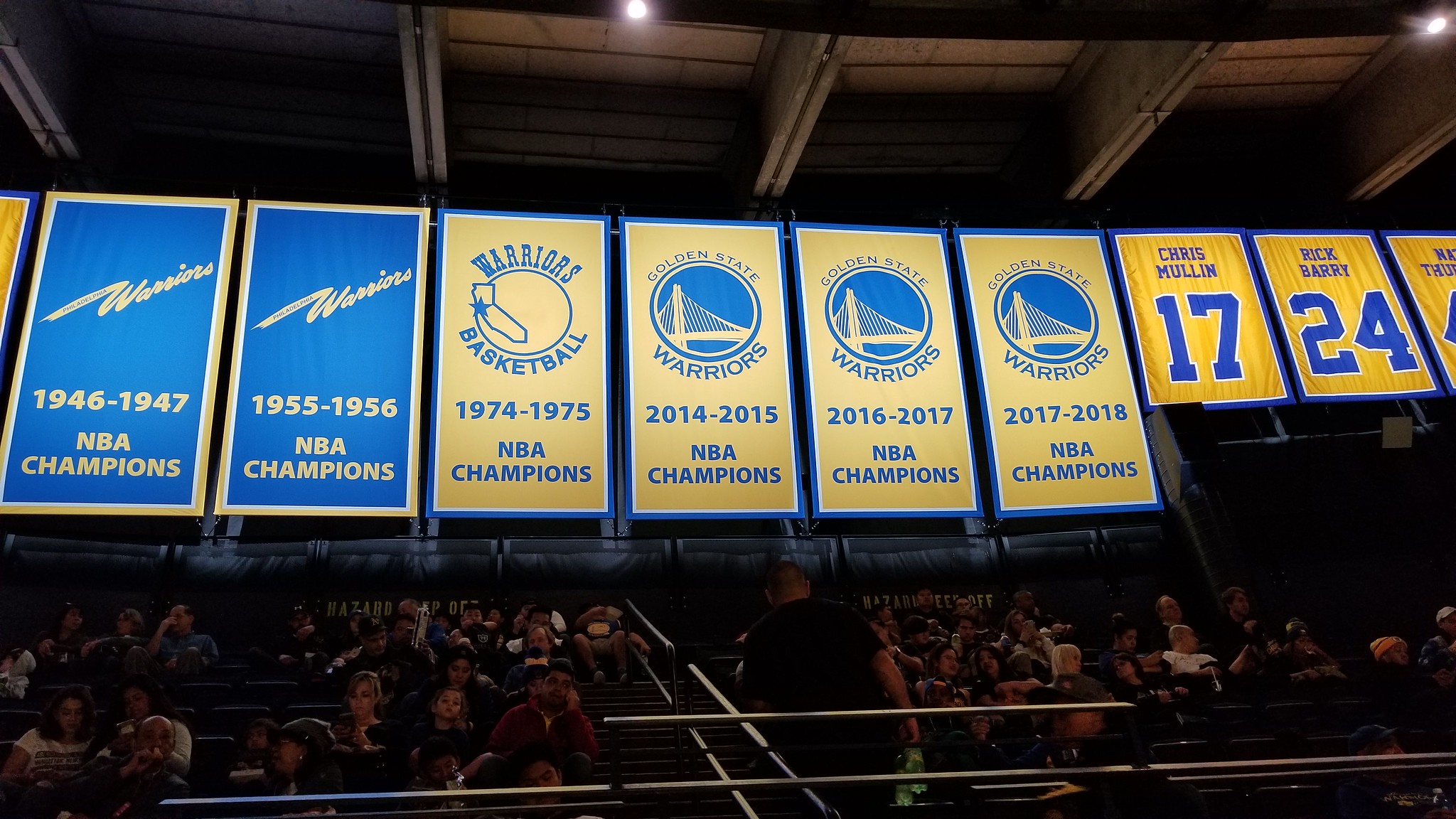This detailed photograph captures an interior view of a stadium, focusing on the back section where spectators are seated in black chairs. A central staircase, bordered with black metal railings, divides the seating area. At the top of the image, near the ceiling, six vertical blue and gold banners line the wall, commemorating the Golden State Warriors' NBA championships with various years inscribed in white or gold lettering, spanning from 1946 to 2018. Adjacent to these championship banners are jersey banners displaying the retired numbers of notable players such as Chris Mullin (#17) and Rick Barry (#24), each designed in yellow with blue accents. The lower portion of the image reveals the word "Hazard" partially visible on the wall behind the seated attendees. The atmosphere appears calm, with attendees seemingly focused on the event, yet not particularly animated with excitement.